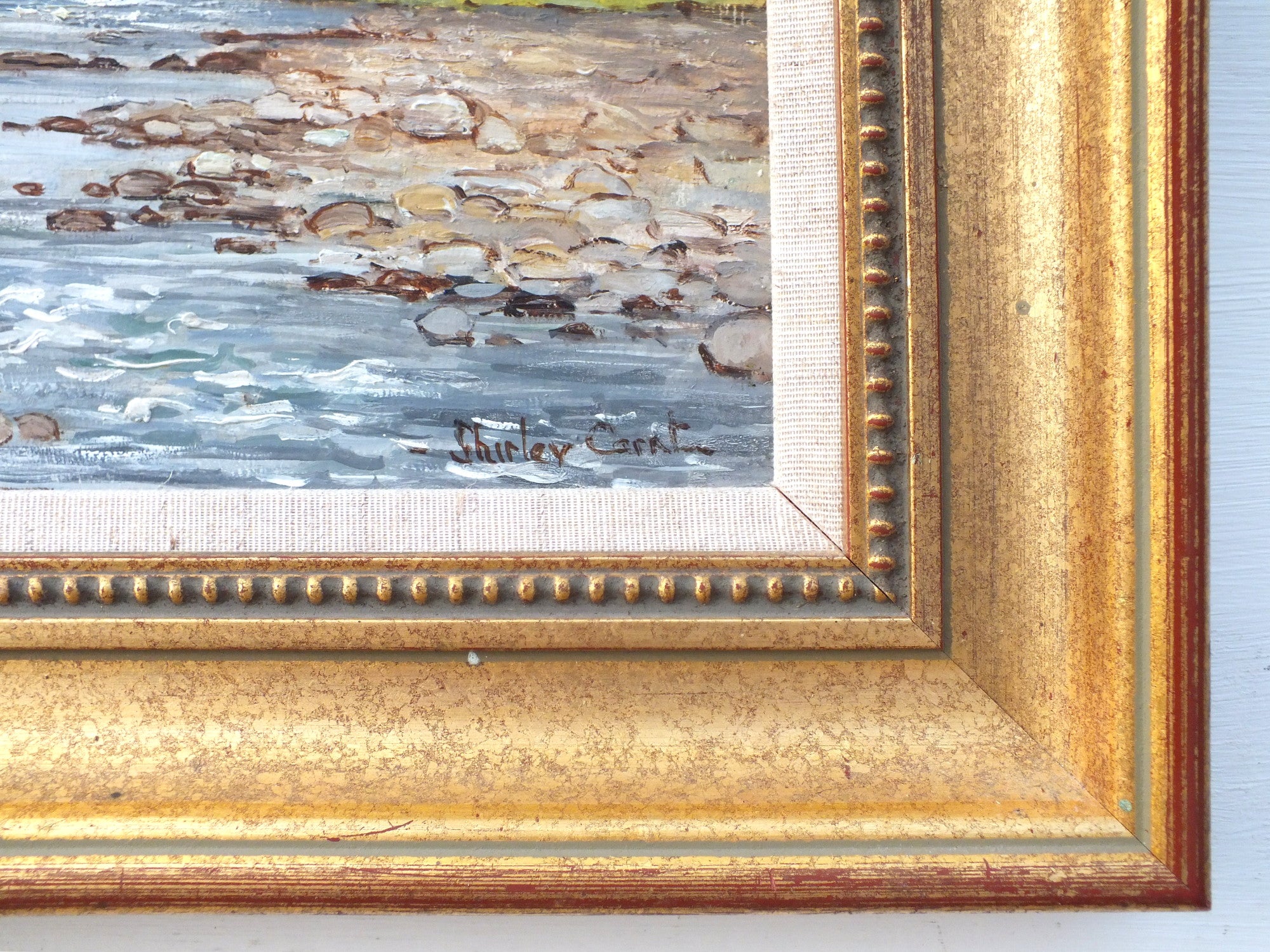This image captures the bottom right corner of a large painting, focusing on detailed elements of both the frame and a section of the artwork. The frame is an elaborate, golden brown with a thick border that features a beveled design. The outer edge of this frame has a reddish-brown tint with golden streaks, while the inner border is adorned with a beaded pattern. Inside the frame, there's a white, textured matting that elegantly borders the watercolor painting itself.

The visible portion of the painting depicts a tranquil water scene; rippled blue water gently touches the shoreline, which is scattered with gray and brown pebbles and rocks. This sliver of the painting showcases various shades of light blue, white, and brown. In the bottom corner of the artwork, the artist’s signature is visible, reading "Shirley C-A-R-N-T..." though the last letters are not clearly discernible. The painting is hung on a blue-colored wall, adding a background hue that complements the artwork's palette.